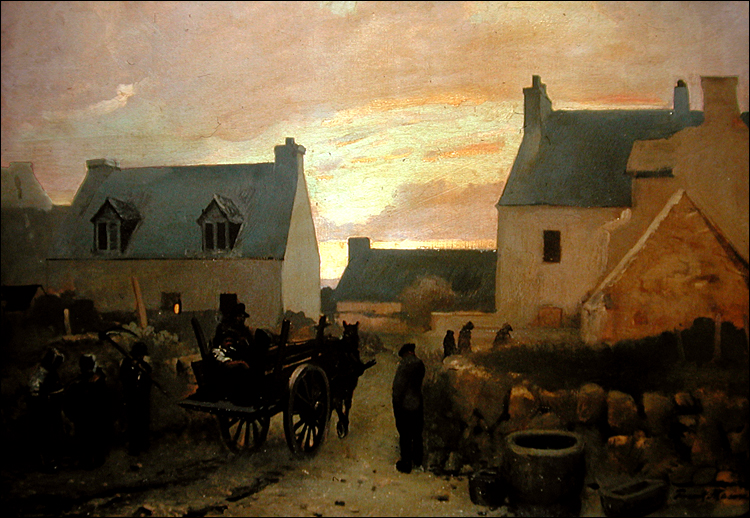The painting captures a serene rural village at the early hours of sunrise or the onset of dusk, enveloped in a wash of warm and cool hues that splendidly depict the sky's transitioning colors. The scene features several small, whitewashed plaster homes, giving an inviting charm to the village. Central to the painting, a horse-drawn, two-wheeled cart is depicted with a man driving it, possibly a private cart or one used by a traveling merchant. The cart seems to be navigating between two prominent houses. The village scene is dotted with other figures, portrayed in black, silhouetted shadows, emphasizing the contrast with the ambient light. A distinctive, low-lying circular rock wall, about five to six feet tall, frames an empty, large barrel outside its perimeter. The dirt road meandering through adds to the rustic feel, while heavy shadows in the foreground provide a dramatic effect, further highlighting the delicate interplay of light and darkness across the painting.